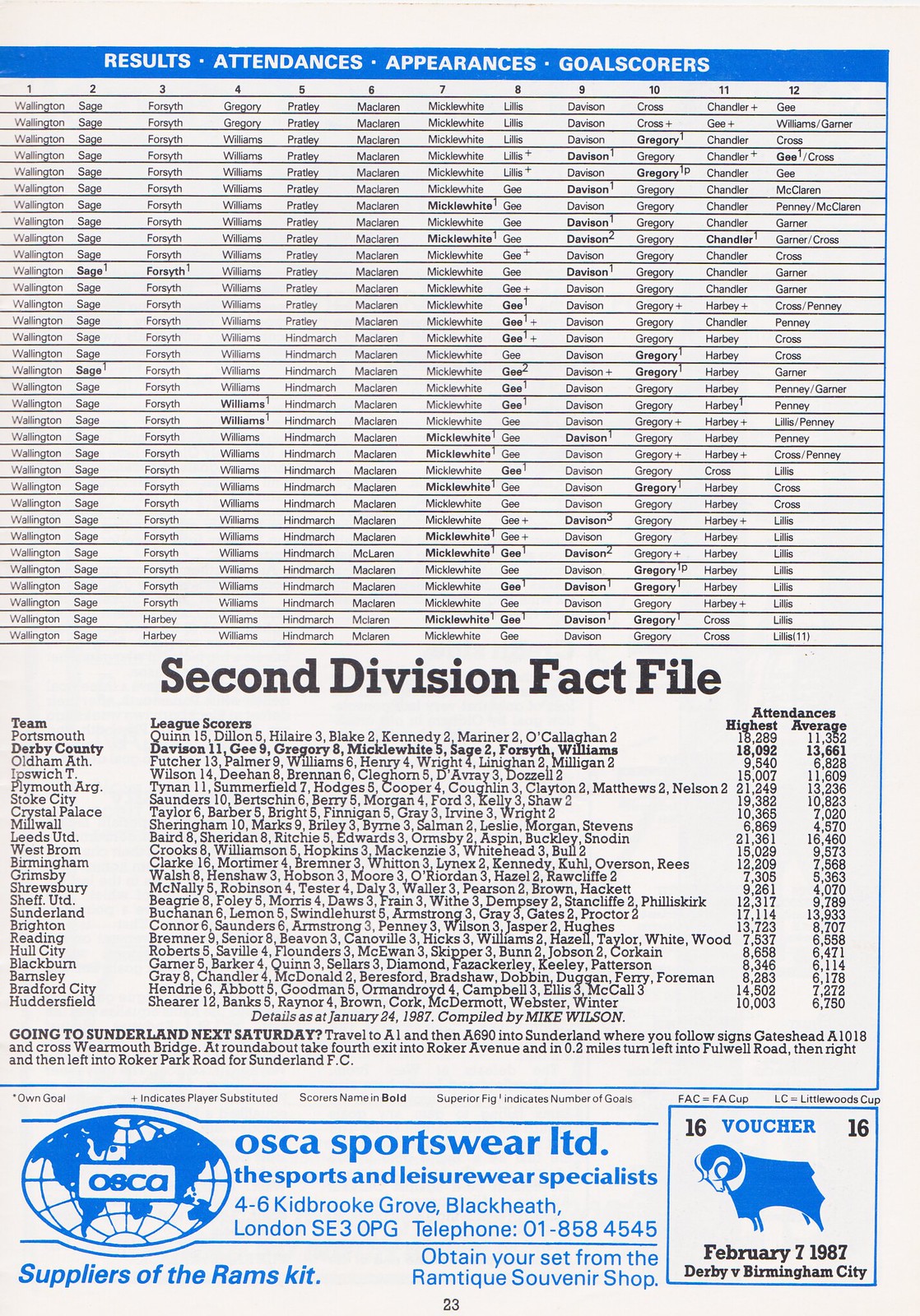This detailed magazine page features comprehensive information, primarily focused on a soccer program. The page is characterized by a blue banner at the top, which prominently displays in white capital letters: "RESULTS, ATTENDANCES, APPEARANCES, GOAL SCORERS." Below this banner is a graph labeled from 1 to 12, running left to right, listing various player names such as Wallington, Sage, Forsyth, Gregory, Williams, Pratley, McLaren, Micklewhite, Lillis, Davis, and others. This pattern of names repeats several times down the page.

The background is white, and in the bottom middle section of the page, the black letters spell out "Second Division Fact File." This section includes details about teams, league scores, and attendance figures, breaking down the highest and average attendances. Additionally, travel directions to an upcoming match in Sunderland and details for attending it are provided, such as the optimal travel route via AI and A890.

Toward the bottom of the page are two advertisements: one for OSCA Sportwear Limited, specializing in sport and leisure wear, and another smaller box highlighting a voucher dated February 7th, 1987, for the Derby versus Birmingham City match.